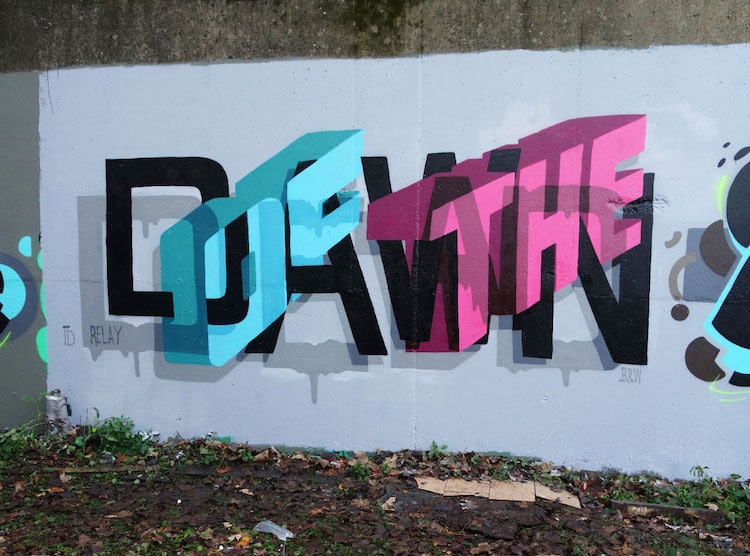This image features a striking mural painted on a concrete wall. The focal point of the artwork is the word "Dawn" rendered in bold black block letters with soft gray shadowing behind them that appears slightly dripping, enhancing the graffiti-like effect. Perpendicular to "Dawn" are the words "Of" and "The," which are vividly colored in cyan and pink, respectively, and depicted in a 3D style that seems to jut out from the wall. These 3D words intersect "Dawn" at an angle extending from the lower left to the upper right. The word "Of" is positioned in a dynamic 3D manner, along with "The," adding depth and complexity to the composition. Moreover, the mural includes an intriguing element: a keyhole-shaped illustration on the right side, partially cropped out of the frame. Below "Dawn" in the lower right corner, the letters "B" and "W" are inscribed. Painted against a primarily white background, the entire mural creates a visually compelling interplay of colors, dimensions, and shadows. Notably, this masterpiece is attributed to the artist TD Relay.